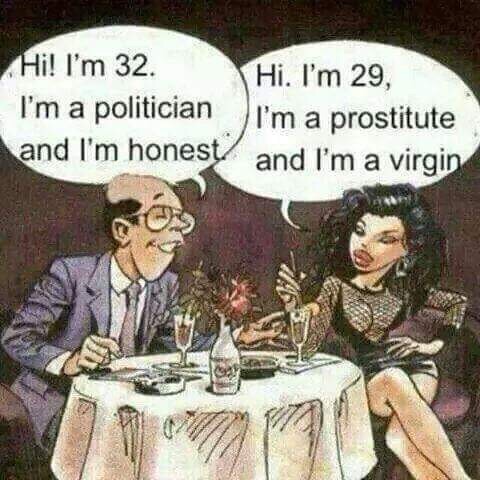The image is a detailed comic drawing depicting a man and a woman conversing at a restaurant, seated around a circular table draped in a white cloth. The man, positioned to the left, introduces himself through a speech bubble, reading, "Hi, I'm 32, I'm a politician, and I'm honest." He is characterized by his balding head, with hair only above his ears and at the back, and he wears glasses. He is dressed in a blue suit paired with a tie and a white undershirt, sporting a sharp nose and a prominent chin, adding to his attempting-to-be-appealing demeanor towards the woman.

The woman, sitting on the right, has a speech bubble stating, "Hi, I'm 29, I'm a prostitute, and I'm a virgin." She has voluminous, curly black hair that poofs out around her head, accented with gray eye shadow over thin eyes. Her puffy lips and seductive attire—a black evening or party dress with cleavage showing and fishnet details on the shoulders and chest—complete her provocative look. She is depicted with crossed legs and is holding a fork with food from a nearby plate.

The scene is set against a dark, purplish-gray or reddish backdrop. The table is adorned not only with their cocktails but also features a white vase with flowers and an ashtray. The overall ambiance suggests an intimate setting where the woman looks interested in the man, while he tries to appear genuine and appealing.